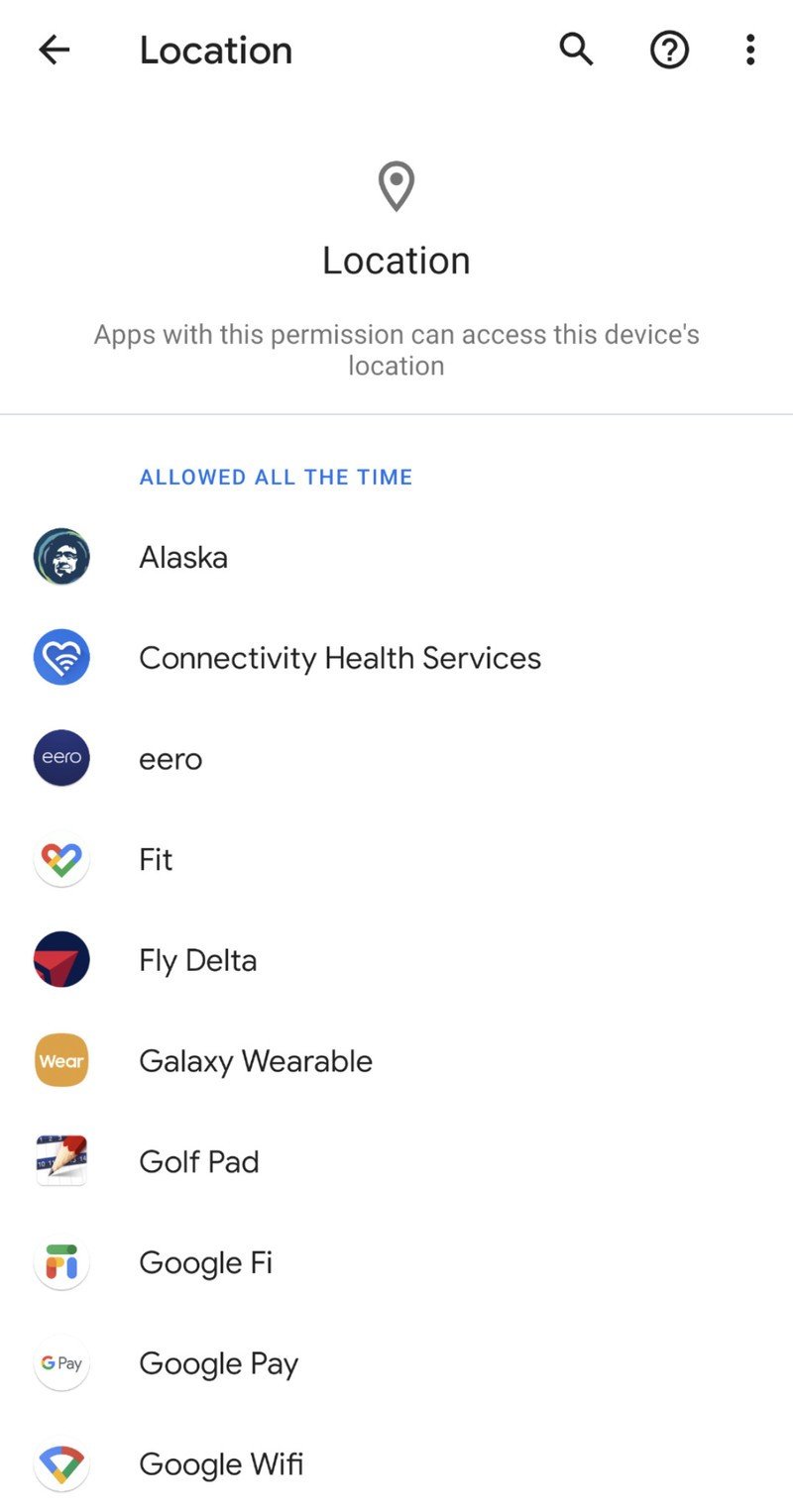Screenshot of a cell phone's location settings. At the top left corner, the word "Locations" is displayed in bold font with a capital "L" and a back arrow to its left. To the right of this title are three icons: a magnifying glass, a question mark inside a circle, and a vertical three-line menu symbol. Directly below, there is a location icon resembling a teardrop with a circle at the top, placed centrally. Below this icon, the word "Location" is displayed, followed by the description "Apps with this permission can access this device's location." Beneath this description, the heading "Allowed all the time" lists the following apps: Alaska, Connectivity Health Services, Aero, Fit, Fly Delta, Galaxy Wearable, Golf Pad, Google Fi, Google Play, and Google Wi-Fi.